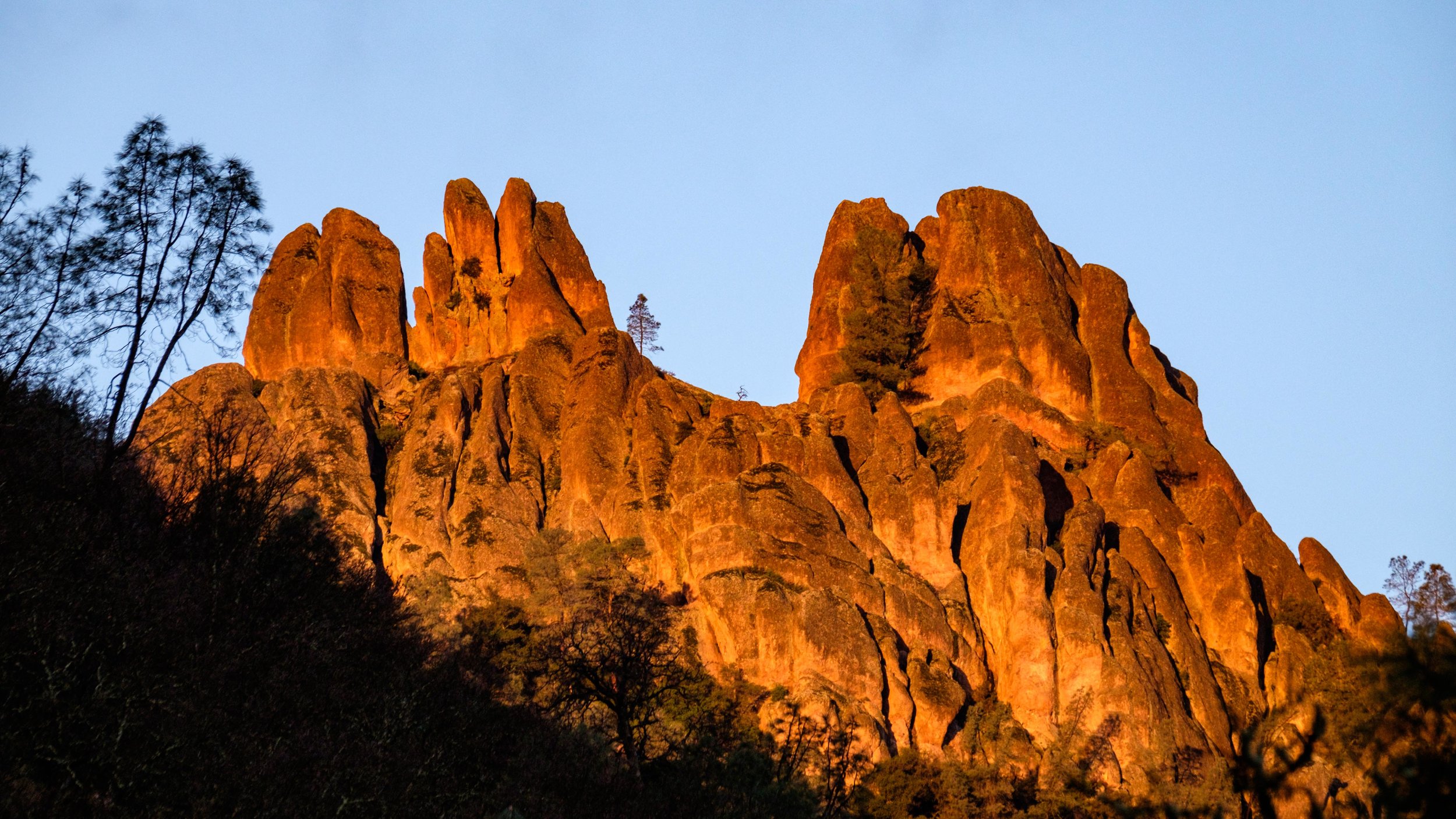This photograph captures a striking desert mountain with distinctive rock formations bathed in the warm hues of sunlight. The mountain, characterized by its steep bluff-like structure, exhibits a palette of earthy browns, reds, and oranges, accentuated by light and shadows that create a dynamic visual effect. The mountain's peaks vary in shape, ending mostly in rounded edges or flat tops rather than jagged points, offering a unique and inviting challenge for hikers.

The formation features notable details such as a pronounced V-shaped gap near its center, with two prominent peaks on the left and one large peak on the right. Small trees and bushes are visible within this gap, appearing diminutive against the towering rocks. The rocky structure is surrounded by sparse vegetation, including evergreen-style trees and dark brush, which appear silhouetted due to the strong sunlight and the early or late hour at which the photo was taken.

In the bottom corners of the image, there are silhouettes of hills, with weedy shrubs and grass adding texture to the foreground. The sky above is a clear, light blue, providing a serene backdrop to the rugged, sunlit mountain. This natural tableau, with its rich colors and intricate rock formations, epitomizes the serene and timeless beauty of desert landscapes.